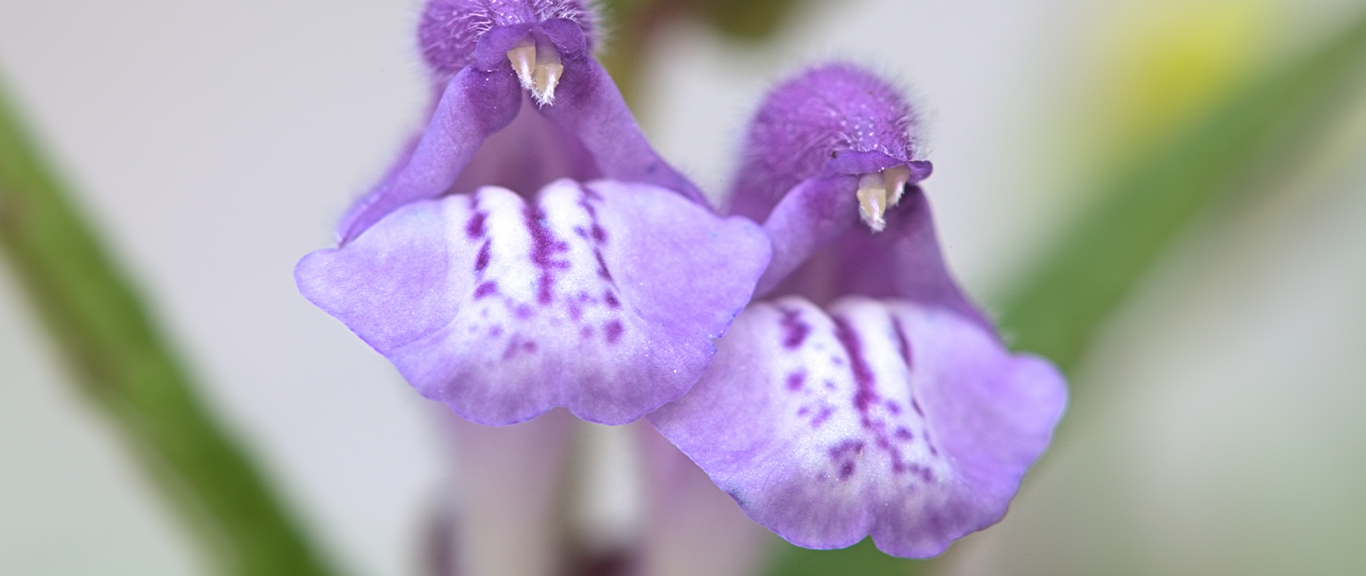This is a remarkably close-up photograph of two unique, purple flowers with striking, almost animal-like characteristics. The flowers, which resemble lady slippers or weeping tulips, feature intricate details that captivate the viewer’s attention. The petals are primarily purple with lighter purple hues on the sides and are adorned with dark purple specks, giving them a spotted appearance. At the very tip of each bloom, two white, tooth-like structures emerge where the pollen is visible, adding to their unusual look. The flowers' surfaces have a fuzzy texture, and you can even see the fine hairs on the blooms. In the background, blurred green branches and leaves with a faint yellow hue create a soft, indistinct backdrop, ensuring that all focus remains on the two closely positioned flowers, which might even be touching. The dew drops on the petals add a touch of natural beauty to this stunning and highly detailed close-up image.